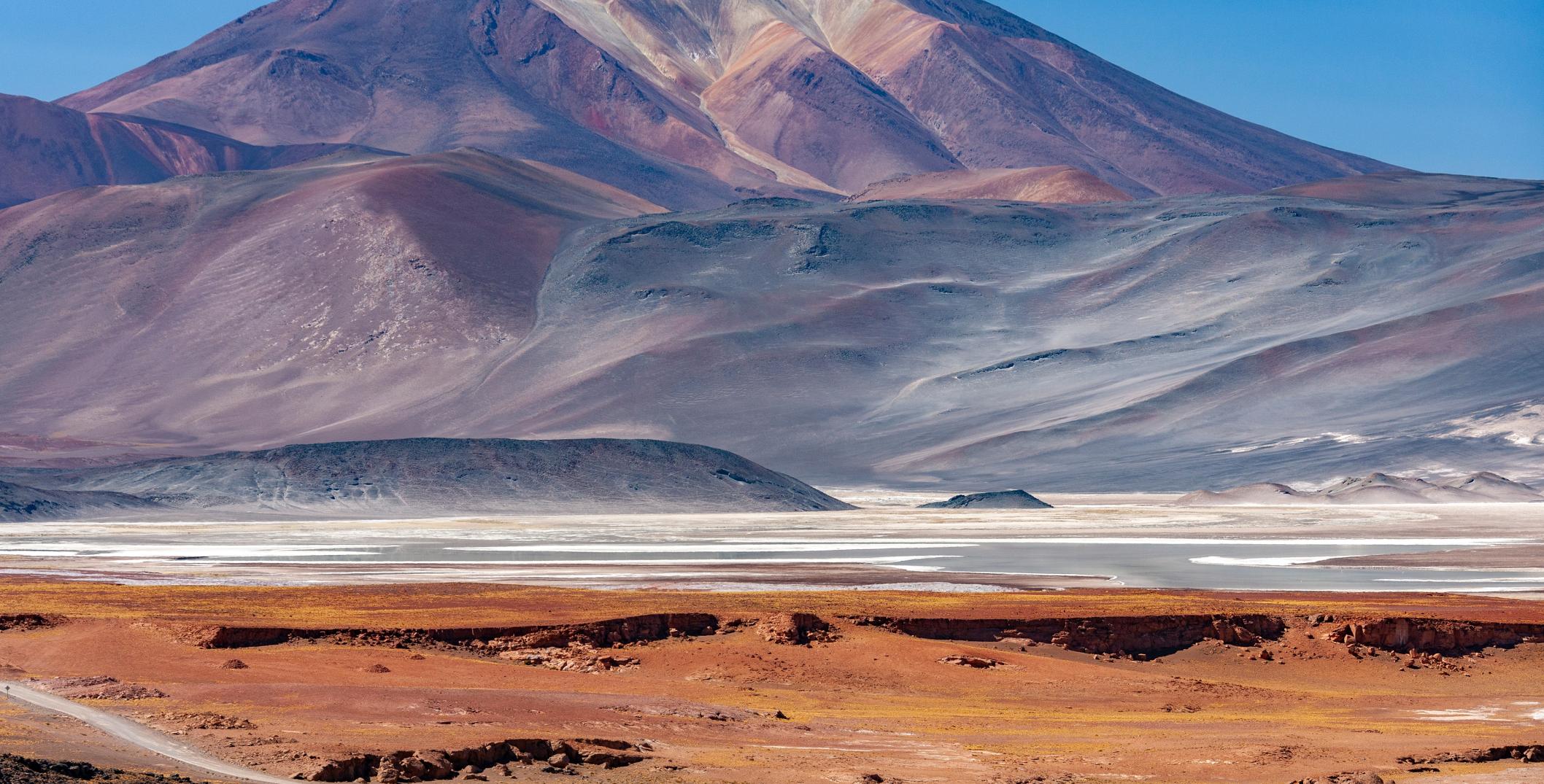The image depicts a breathtaking, horizontal panoramic nature scene characterized by a massive, awe-inspiring mountain as its main focus. The mountain's surface is rocky and rugged, devoid of greenery, with striking patches that transition from light to dark, creating dramatic shadows. The peak is not visible, adding to the mountain's imposing presence. Behind this giant natural structure, a perfect blue sky stretches across the backdrop.

In the foreground, the terrain is predominantly red clay, with subtle streaks of yellow interspersed among the burnt orange ground. This foreground area is reminiscent of a prairie or desert landscape, lacking in grass or greenery. There is a notable white strip running diagonally across the bottom left, appearing to be a road, which is light gray in color.

Further back, there are areas that resemble a salt flat, featuring very white, almost grayish terrain that contrasts with the more colorful foreground. This expansive landscape transitions smoothly into the base of the mountain, which then rises steeply, becoming more massive and sheer as it ascends. The mountain itself displays a stunning array of colors, including dark red, orange, brown, gray, and even hints of light blue and teal, enhancing its majestic and grandiose appearance.